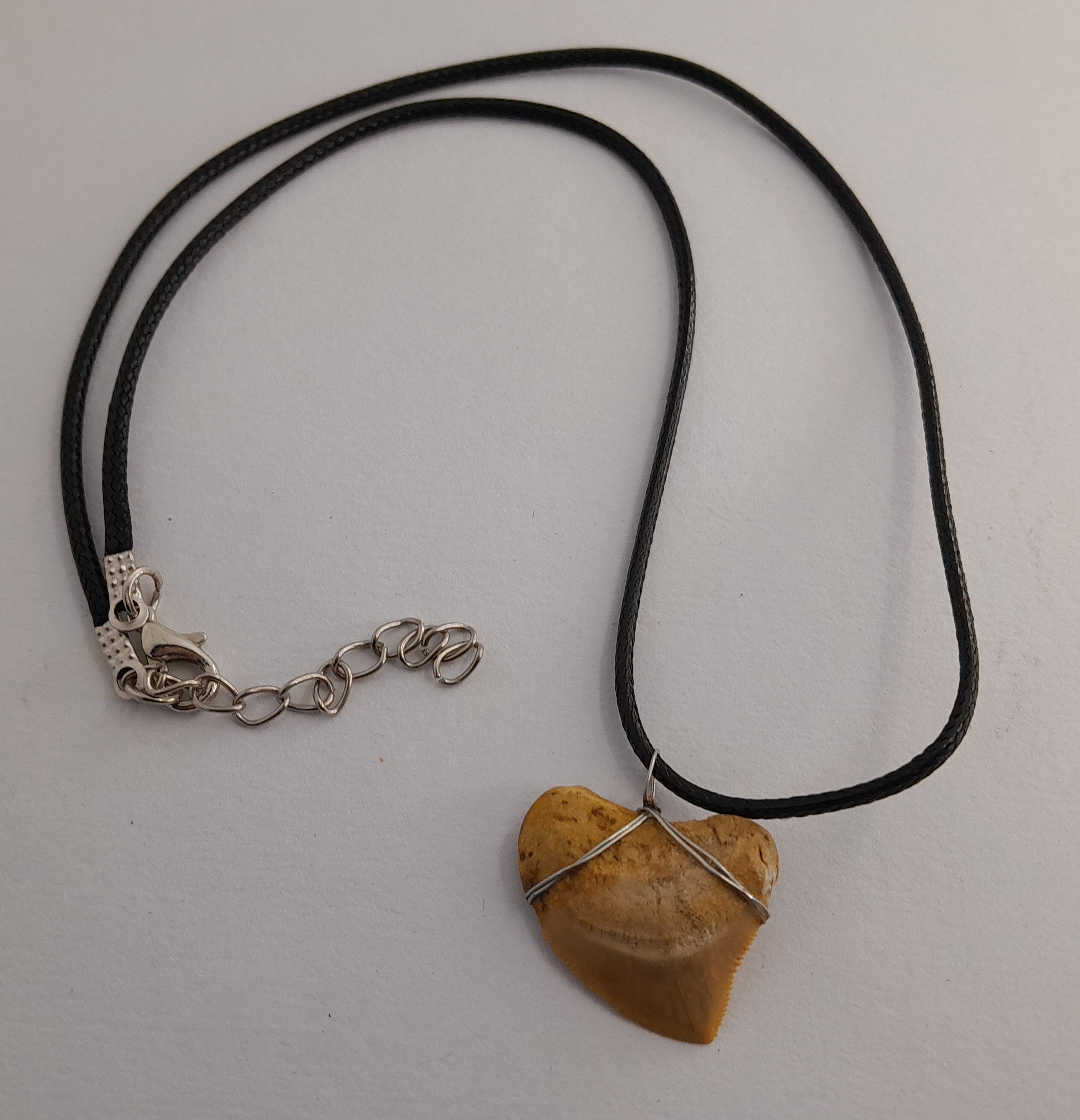This close-up photograph showcases a unique necklace displayed against a whitish-gray background. The centerpiece of the necklace is a broad, fat, heart-shaped rock of rich brown color, which resembles a prehistoric tooth due to its serrated edges. The rock is securely wrapped with silver wire at its top, mimicking where roots would connect to gums, adding a rustic charm to the piece. This centerpiece is suspended from a black ribbon-style necklace, which is integrated with a thin silver chain for added elegance. The necklace features a lobster claw clasp in a matching silver color, ensuring it stays securely fastened around the neck. The entire setup is intricately detailed, highlighting both the natural beauty of the rock and the craftsmanship of the wire wrapping and necklace design.